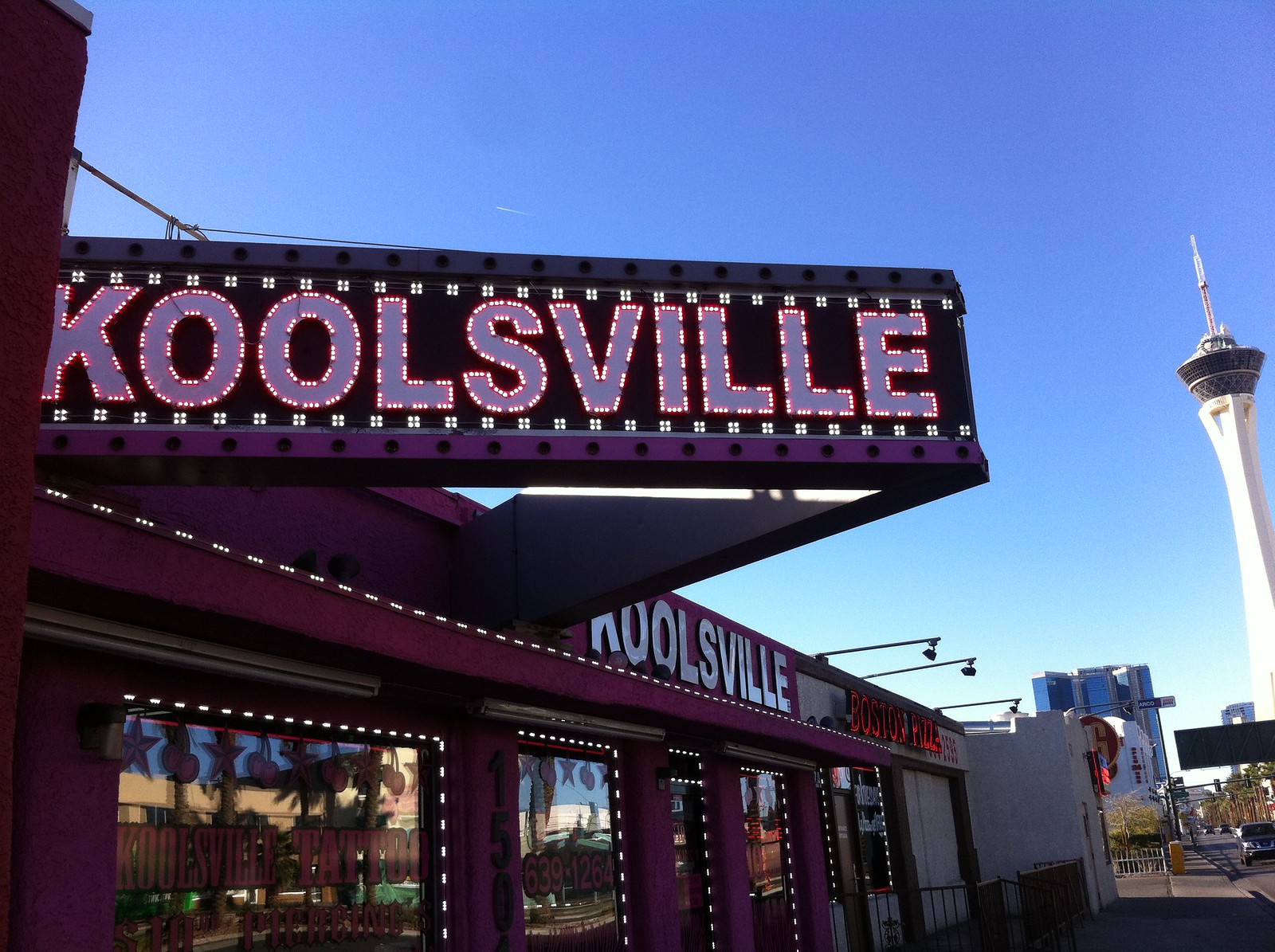The photo captures a vibrant street scene in what appears to be Las Vegas. Dominating the image is a row of storefronts, with the most prominent being a tattoo parlor named "Coolsville," which is spelled with a "K" instead of a "C". The building housing Coolsville is painted in shades of dark pink or magenta, and its marquee is outlined in lights, featuring the name "Coolsville" in pink text. Adjacent to it is another storefront with red text on a white facade, possibly a pizza place named Boston Pizza. The setting includes a clear sky with no clouds, subtly marked by the faint trail of a jet above the Coolsville marquee. In the background, the iconic Stratosphere tower stands tall with its white structure accented by black and blue at the top, adding a distinctive Vegas skyline touch. The street in front of the buildings is active, with cars in motion, capturing the lively atmosphere of the area.